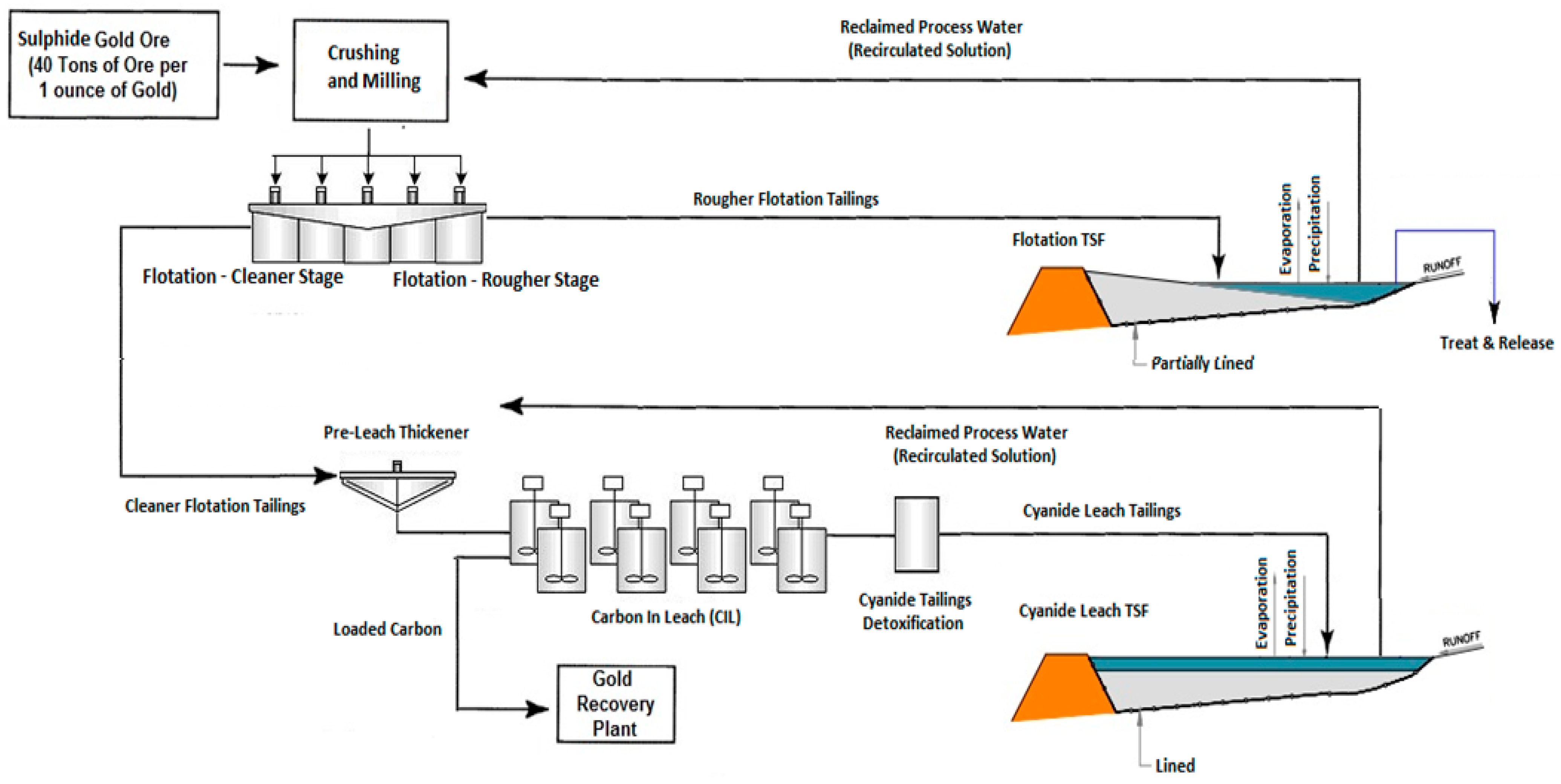This detailed diagram illustrates an industrial gold processing system, presented with black text on a white background. At the top left, the process begins with "Reclaimed Process Water (Recirculated Solution)" and "Sulphide Gold Ore (40 tons of ore per 1 ounce of gold)." Arrows guide through various stages, starting with "Crushing and Milling" and continuing with series of steps involving specialized equipment and processes.

A prominent colorized section, depicted in orange, gray, and blue, labeled "Evaporation, Precipitation, Partially Lined Flotation TSF," features arrows leading to and from it, marked "Rougher Flotation Tailings." Below this section, the diagram shows containers resembling batteries with antennas, representing different flotation stages: "Flotation Rougher Stage" and "Flotation Cleaner Stage."

Further down, arrows lead to a "Pre-Leach Thickener," followed by "Cleaner Flotation Tailings" which direct into a sequence of "Carbon in Leach" silver squares. These squares exhibit lines with small circular elements, moving toward "Cyanide Tailings Detoxification" and "Cyanide Leach Tailings." The arrows transition to "Cyanide Leach TSF," eventually concluding at the "Gold Recovery Plant."

The layout is intricate, with multiple arrows delineating connections between processes like evaporation, runoff, and detoxification, emphasizing the cyclic and detailed nature of gold extraction and water reclamation within an industrial framework.